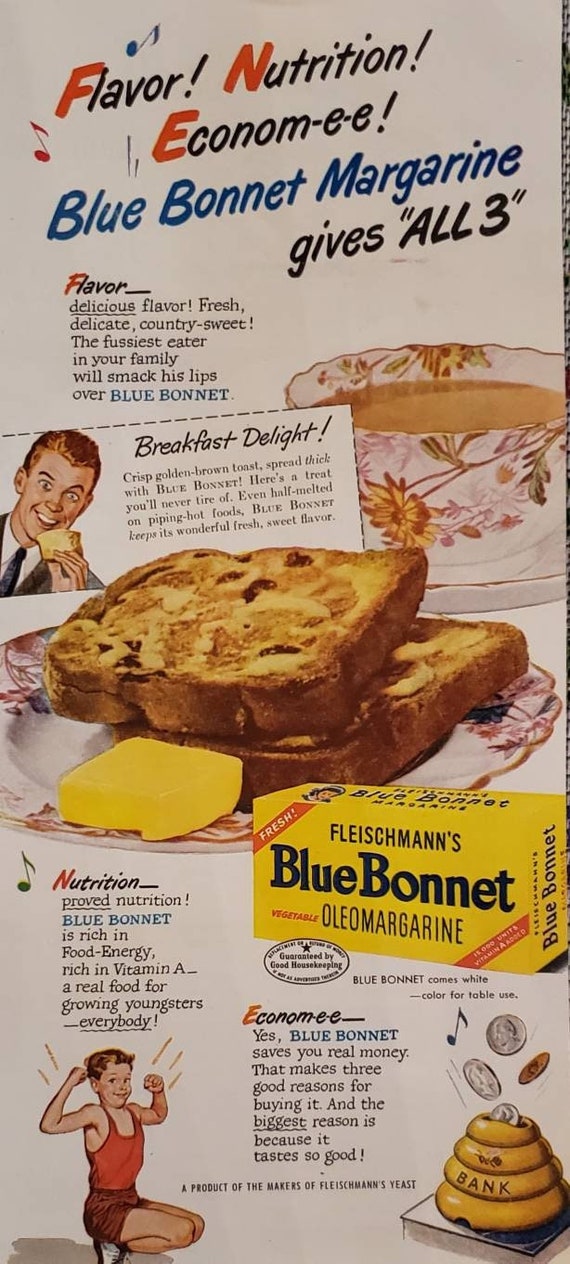This vintage advertisement for Fleischmann's Blue Bonnet Oleo Margarine exudes charm and nostalgia, likely originating from the 1940s or 1950s. At the top, it prominently showcases a jingle with music notes, "Flavor, Nutrition, Economy, Blue Bonnet Margarine gives all three," encapsulating the product's key benefits. Below the jingle, the text elaborates on each benefit—highlighting the margarine's delicious, fresh, and country-sweet flavor, its nutritional value, and its economic advantage.

Central to the advertisement is an artistic and colorful illustration featuring a breakfast setting. A boy, depicted in cartoon style, holds a piece of margarine, accompanied by the label "Breakfast Delight." Nearby, a cup of tea and an ornate plate with two slices of toast, each adorned with a pat of Blue Bonnet margarine, complete the appetizing scene.

On the bottom left, another boy is shown flexing his muscles, symbolizing the nutritional benefits of Blue Bonnet margarine. To the right, a piggy bank with coins falling into it indicates the product's cost-effectiveness, reinforced by the text suggesting significant savings for families.

The advertisement is richly detailed with vibrant illustrations and period-specific aesthetics that evoke a bygone era while making a strong case for why Blue Bonnet Margarine is a must-have for flavor, nutrition, and economy.